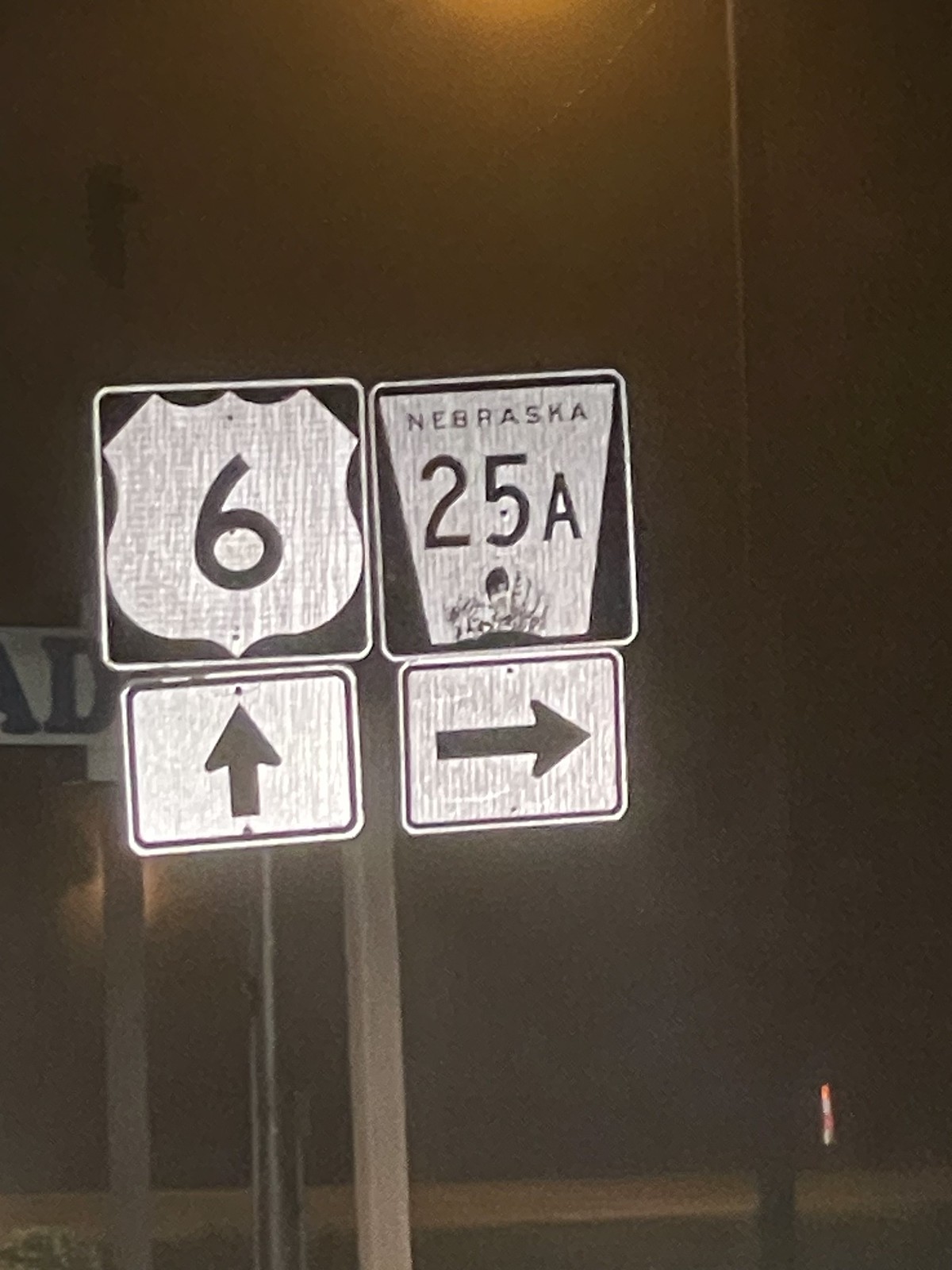In this night-time photograph, the scene is illuminated by artificial light, likely from a camera flash. Dominating the top of the image is the diffuse glow of a streetlight positioned over a highway intersection. A highway sign mounted on a slightly leaning single post is prominently featured, clearly indicating directions for Highway 6 and Nebraska 25A. The sign shows that continuing straight ahead keeps you on Highway 6, while a right turn leads toward 25A. In the foggy and mist-covered background, another sign is just visible, though its details are obscured by low visibility and lack of illumination. The bottom of the image reveals a portion of the road running horizontally from left to right, which intersects with the path leading to Nebraska 25A.